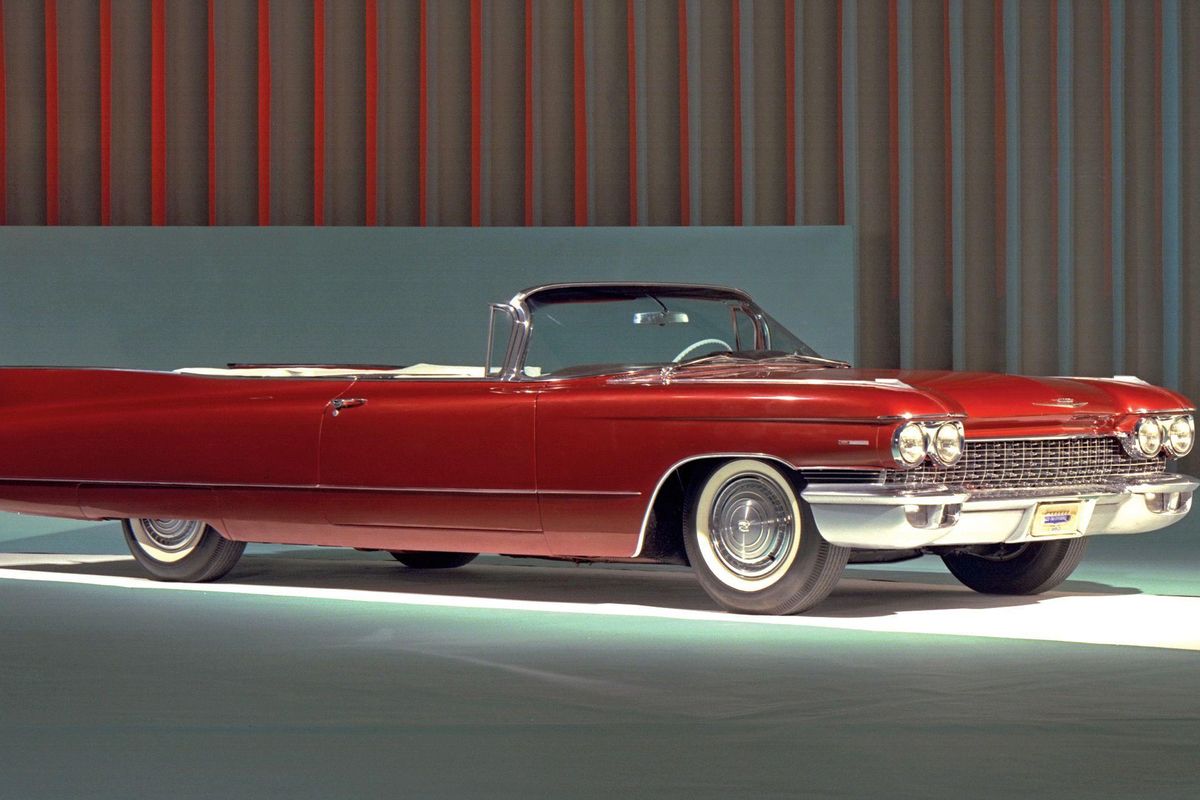This is a detailed photograph of a retro convertible car with an unmistakably classic design. The bright yet dark red vehicle is oriented towards the right side of the image, with the front of the car nearly touching the right edge and the rear slightly extending beyond the left edge. The car is characterized by its extended length and low riding profile, featuring prominent silver accents and a sleek glass windshield. The convertible top is retracted, revealing a white steering wheel and a hint of a white top near the back of the car.

The front of the vehicle is marked by a chrome bumper and four distinctive headlights. The car's four wheels are visible, with the front tires fully exposed and the rear tires partially covered by the car's body, almost touching the ground.

The setting of the photograph is somewhat ambiguous - it could either be an interior showroom or a large warehouse, as there are no defining details to confirm the location. The car is positioned on a blue-gray and white flat surface, parked in front of a wall that is a mix of solid gray sections and vertical lines in tan, gray, and red. The wall appears to be illuminated by blue and red lights, possibly contributing to a red-tinted appearance of the backdrop. There are no people or text visible in the image, drawing full attention to the striking details of the vintage car.